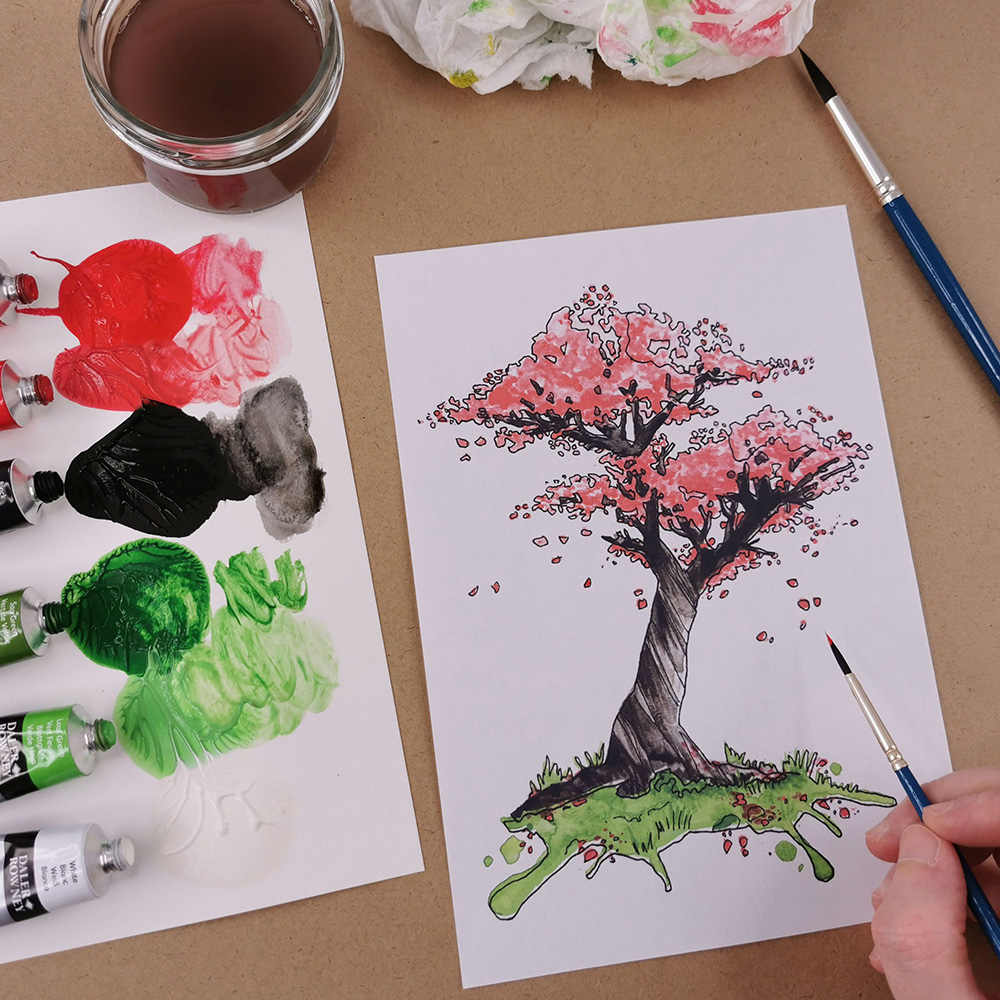This image offers a detailed view from the perspective of an artist engrossed in painting a delicate cherry blossom tree. The artwork, painted on a rectangular piece of white paper, depicts a twisted, dark gray and black trunk with pink and red blossoms. The tree sits atop a patch of green grass, created with a splattering technique. The scene is devoid of a sky backdrop, leaving the white paper as the background.

On the left side of the image, six tubes of paint are laid out on a sheet of paper, each with a dab of paint squeezed out in front of it. The paint colors include dark red, reddish pink, dusty red, black, dark green, light green, and white. At the top left, a circular container filled with dirty, brownish water is visible – likely used for rinsing brushes. In the top middle, a crumpled paper towel stained with various paint colors can be seen, while at the top right, another paintbrush rests.

The artist's hand, appearing in the lower right corner, holds a fine-tipped paintbrush with a blue handle and silver ferrule. The painting appears to be set against a light brown wooden surface, adding warmth to the creative scene. Overall, the image captures the intricate process of creating a hand-painted card featuring a picturesque cherry blossom tree.